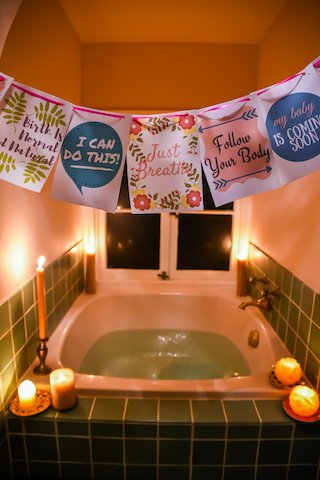The image depicts a large, oval-shaped bathtub surrounded by dark green tiles and is partially filled with water. The atmosphere is serene and inviting, with the tub being encircled by a total of seven lit candles—three taller candles and four smaller ones—which provide a gentle, flickering light. The bathtub's white, and it features a golden faucet, with water that has a serene, light green hue.

Above the tub, there's a series of inspiring banners strung across the ceiling, displaying motivational phrases such as "I can do this," "Just breathe," "Follow your body," "Birth is normal and natural," and "My baby is coming soon," suggesting a therapeutic, preparatory environment for childbirth. The white walls above the green tiles give the space a clean and calming feel, while the couple of windows at the end of the tub, without curtains, allow natural light to filter in, though they might benefit from shades for additional privacy. The overall setting suggests a peaceful, supportive ambiance, ideal for relaxation and mental preparation for an impending birth.